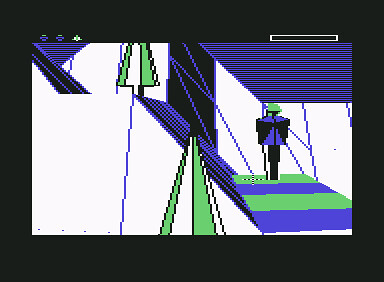The image appears to be a retro pixel art creation reminiscent of early computer graphics. Dominated by shades of blue, green, black, and white, it features a stick-figure-like character. The figure, drawn with black and blue pixelated clothing and wearing a small green helmet or hat, stands on a horizontally striped green and blue platform. This platform is held up by blue wires or ropes, suggesting a suspended structure. Above the character is a blue canopy, with additional blue elements and angular pieces seen in the top-left corner. To the top right, a white bar filled with black is visible. The character appears to be in an ambiguous setting with some green and white elements that could resemble trees or mountains. The entire scene is framed by a wide black border.